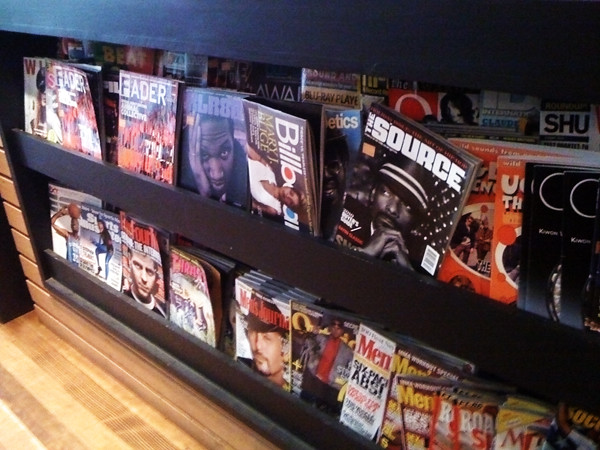The image captures two wooden magazine stands with a total of four shelves, divided by a sleek black wooden partition. These stands are situated indoors, possibly within a bookstore or a magazine shop, evidenced by the orderly arrangement and diverse selection of magazines. The light wooden planked floor visible in the bottom-left corner adds to the cozy indoor setting. 

Each stand features two rows of magazines, illuminated gently by natural light coming in from the left side of the frame. The magazines, stacked both behind and below the horizontal black bar that runs along the shelves, showcase their readable covers prominently. Titles like "Fader," "Billboard," "The Source," "Men's Health," "442," "Men's Journal," and "Shoe (S-H-U)" are visibly arranged in a vibrant display of colorful covers. Celebrities and various themes adorn the fronts, indicating the magazines cover a broad spectrum of interests, including sports and men's lifestyle. The detailed organization and variety suggest a well-stocked and inviting place for browsing.